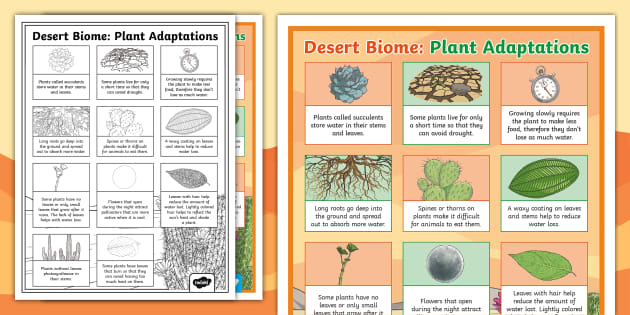The image depicts a page from a children's workbook focusing on desert biome plant adaptations. On the right-hand side, the page is in full color, with "Desert Biome" written in red outlined in white, and "Plant Adaptations" in green outlined in white. Below these titles is a 3x3 grid of illustrations against an alternating orange and yellow background. Each illustration is accompanied by a white box with black text explaining various plant adaptations. Examples include a stopwatch icon with the text, "Growing slowly requires the plant to make less food, therefore they don't lose as much water," and an illustration of succulents stating, "Plants called succulents store water in their stems and leaves." 

On the left side of the image, there is a black-and-white version of the same page, positioned to the left of and slightly overlapping with the colored page. This black-and-white page appears to be an exact duplicate but rendered without any color, giving it a more straightforward, outline-based appearance. Both pages highlight the same key adaptations, including plants that avoid drought by living for only short periods and those that grow slowly to conserve water. The color page seems to be a close-up as it only displays the top half, making nine of the total illustrations visible while the left side hints there might be more beyond what is shown.